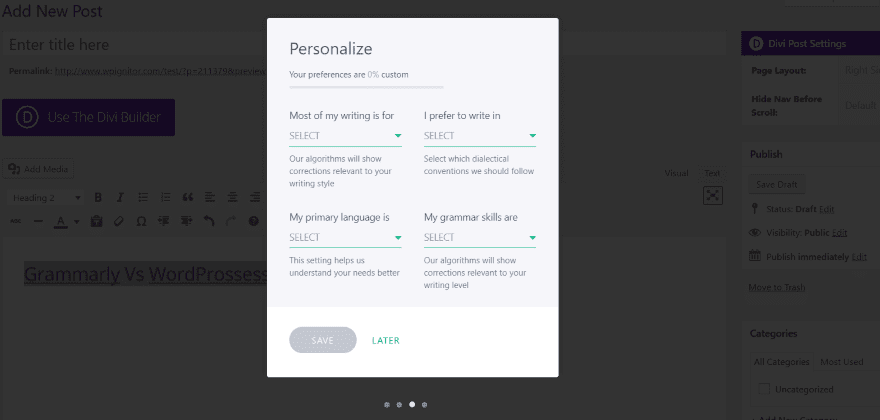The image depicts a computer screen displaying a grayed-out website or program interface, interrupted by a large pop-up window occupying about half of the screen. The pop-up window features a white background with black lettering and includes four dot navigation indicators at the bottom, with the third dot currently active.

At the top of the pop-up, the title "Personalize" is prominently displayed. Below this, the text indicates that "your preferences are 0% custom," followed by a progress line. The main content of the pop-up is divided into a series of two-column rows with selectable options:

1. The first row reads "Most of my writing is for" with a blue "Select" drop-down menu next to it. Underneath, it states, "Our algorithms will show corrections relevant to your writing style."
   
2. The next row states "I prefer to write in" alongside another blue "Select" drop-down menu, followed by the note, "Select which dialectical conventions we should follow."

3. The subsequent row says "My primary language is" with a blue "Select" drop-down menu, explaining, "This setting helps us understand your needs better."

4. The final row reads "My grammar skills are" next to yet another drop-down menu, with the note, "Our algorithms will show corrections relevant to your writing level."

At the bottom of the pop-up are two interactive elements: a gray "Save" button and a blue "Later" hyperlink.